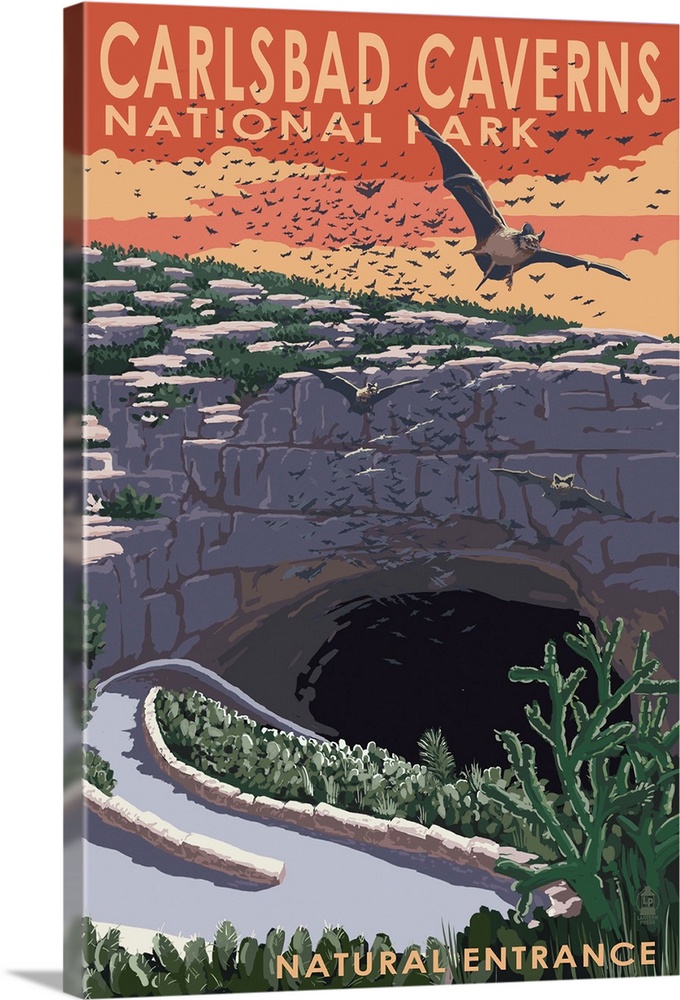This vertically oriented artwork serves as an advertisement for Carlsbad Caverns National Park, showcasing a vivid, painted scene. At the top, the title "Carlsbad Caverns National Park" is displayed in bold white letters set against an orangish sky. Below the title, a multitude of bats are depicted in flight, with one prominent bat in the foreground. The image focuses on a rocky hillside leading down to a large, dark cave—the natural entrance to the caverns—highlighted by the words "Natural Entrance" at the bottom. A winding concrete walkway, flanked by green cacti and bordered by a concrete barrier, guides visitors to the cavern's entrance. The painted artwork captures the rugged gray and granite textures of the rock formation, contrasting with the lively motion of the bats, creating a dynamic and inviting representation of the park.